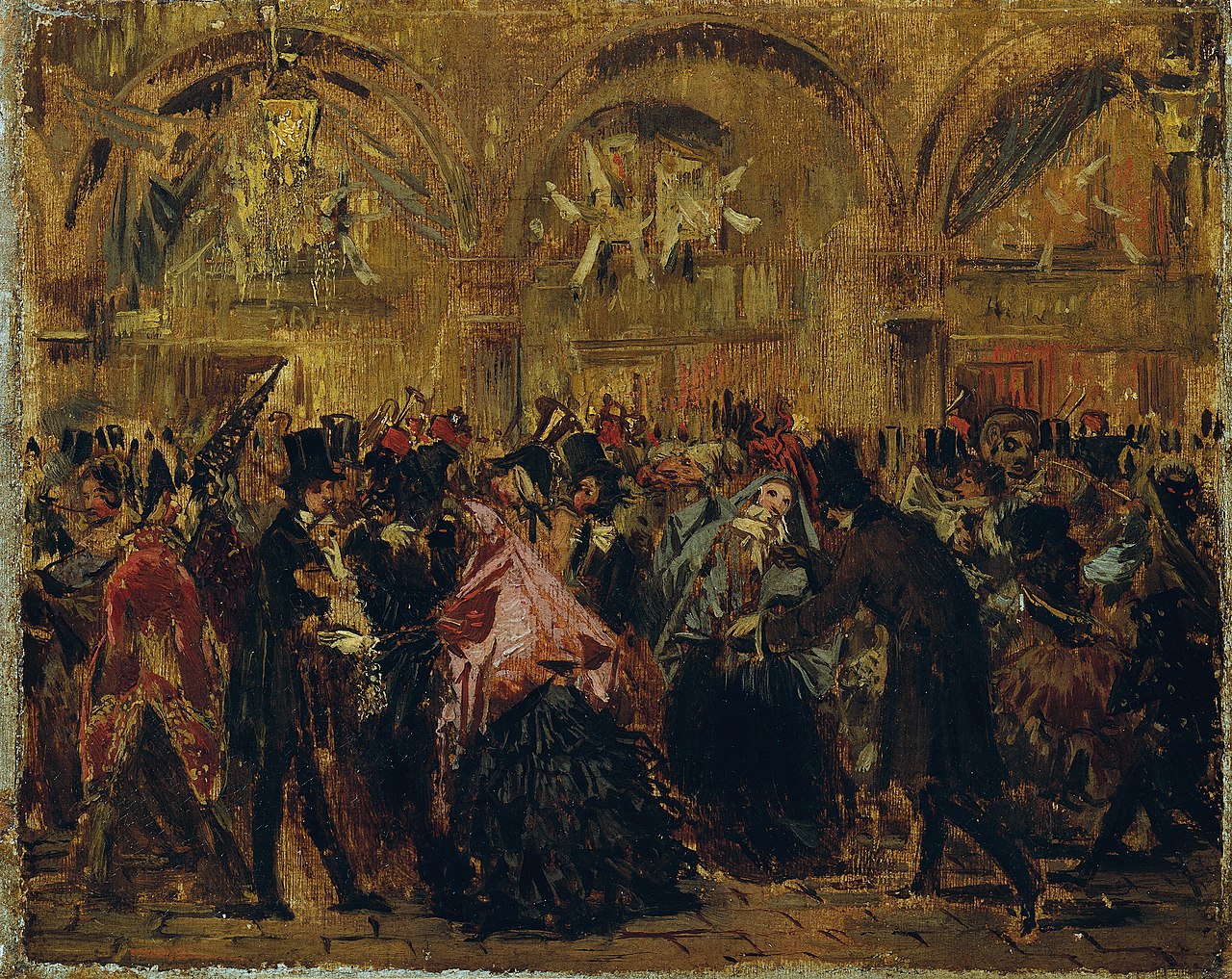The painting vividly depicts a grand, medieval or Victorian-style ballroom filled with around 30 to 100 elegantly dressed figures, dancing and socializing in a celebratory atmosphere. The scene is dominated by a rich golden brown color palette, particularly noticeable on the ornate, high-ceilinged walls adorned with rounded trestles and possibly golden wallpaper. Men in ubiquitous dark top hats and black suits mingle with women in long dresses and colorful scarves, with one woman in a bright pink shawl standing out prominently in the foreground. The intricate details of the attire and the slightly abstract, sometimes inhuman facial features of certain figures add an intriguing layer of mystique to the artwork, enhancing its vintage and historical feel.